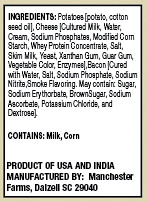This is a detailed image of a rectangular food ingredients label. The label is approximately twice as tall as it is wide, with dimensions around two inches tall and one and a half inches wide. The label features a light yellow (beige) border surrounding a smaller thin black frame, containing the main text area. The background color within the black frame is white, and the text is printed in black ink. 

At the top of the label, the word "Ingredients" is prominently bolded. The actual list of ingredients is printed in a finer, more difficult-to-read print. The main ingredients include potatoes, cottonseed oil, and cheese, with further details specifying components such as cultured milk, water, cream, sodium phosphates, modified corn starch, whey protein concentrate, salt, skim milk, yeast, xanthan gum, guar gum, vegetable color, and enzymes. Additionally, the label lists bacon cured with water, salt, sodium phosphate, sodium nitrate, and smoke flavoring. Possible additional ingredients include sugar, sodium erythrobate, brown sugar, sodium ascorbate, potassium chloride, and dextrose.

The label also highlights that the product contains milk and corn, with "Contains milk and corn" being emphasized in bold print. At the bottom of the label, it notes the product is a "Product of USA and India" and is manufactured by Manchester Farms, located in Dalzell, South Carolina, with the zip code 29040. The overall presentation and the list of ingredients suggest it is a potato-based food product.